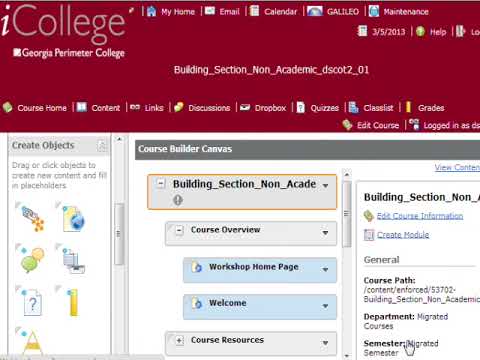The image displays a screenshot of a very old computer interface, likely from the 1990s or early 2000s, seen on a college academic board intended for creating a discussion post. The colors are nostalgic with red, yellow, blue, gray, green, and a touch of maroon. The pop-up window has a label at the top that reads "New Discussion, Building Section Non-Academic, DSC OT 2-01, Georgia Perimeter College" and features a red close button in the top right corner. The central square box shows the interface for writing a forum post, with sections titled "General," "Title," and "Description," where "Open Forum" is the current content. Below these sections, there are interactive GUI icons, along with drop-down menus for categorizing and grading the discussion post, and options for allowing anonymous messages. Additional fields exist but are out of view, as the window can scroll. The bottom of the window has "Cancel" and "Create" buttons. Icons, a mouse pointer, and an overall old-school design emphasize the age of the application.